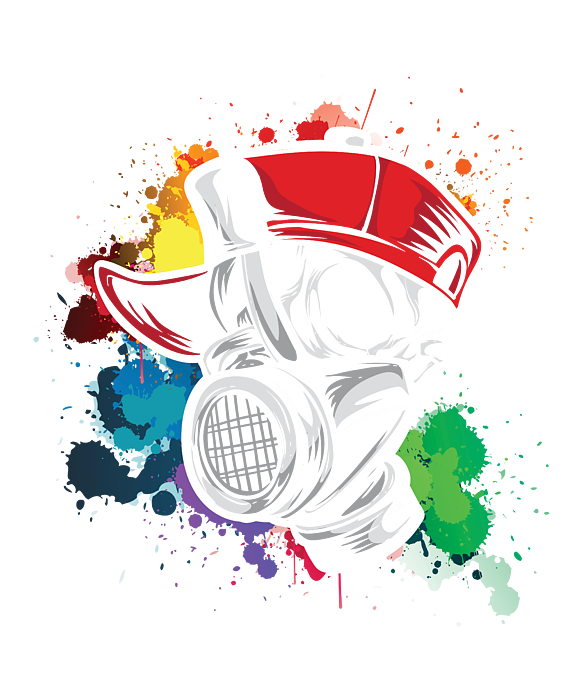The image appears to be a computer-generated impressionist artwork depicting a gas mask with human-like features, adorned with a red and white cap turned sideways with the bill facing left. The gas mask, illustrated in shades of gray, white, and black, consists of intricate details including a central vent and multiple breathing tubes, with one tube extending to the left and another pointing down to the right. The mask's neck area resembles a threaded component, adding an industrial touch to the design. The background is a chaotic array of vibrant paint splashes, featuring a spectrum of colors arranged in a counterclockwise pattern: red and pink at the top, transitioning to orange, yellow, blue, violet, and green splatters towards the bottom and right. The entire scene is set against a white backdrop, enhancing the vividness of the paint colors and the starkness of the mask.